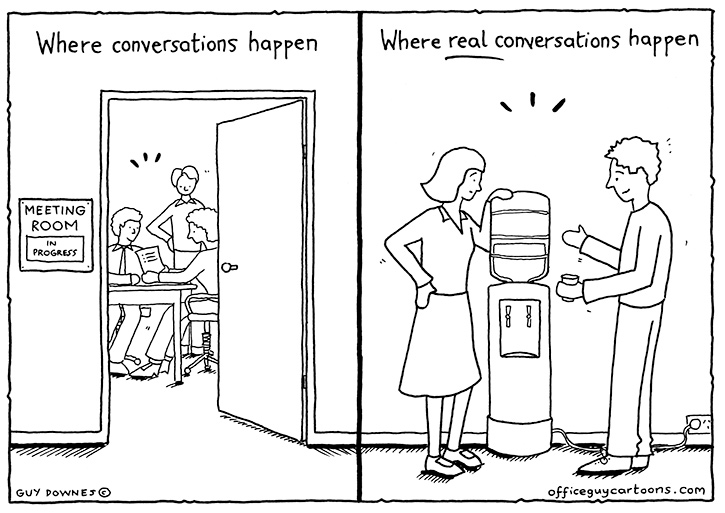This black-and-white cartoon illustration by Guy Downes is divided into two side-by-side panels, each depicting different settings for conversations. 

The left panel, titled "Where Conversations Happen," shows a meeting room in progress. The door to the room is open, revealing a sign that reads "Meeting Room in Progress." Inside, three people are gathered around a table, deeply engaged in discussion. One woman is holding a piece of paper while the other participants have speech lines indicating they are talking.

In contrast, the right panel is titled "Where Real Conversations Happen," with the word "real" underlined for emphasis. It depicts a more informal setting by a water cooler with the classic office water jug. A woman stands on the left side with her hand leaning against the cooler, while a man on the right side gestures animatedly, holding a cup of water. They are clearly engaged in a lively, possibly personal, conversation. 

At the bottom of the panels, the cartoon credits are displayed: "Guy Downes" on the bottom left of the left panel and "OfficeGuyCartoons.com" on the bottom right of the right panel.